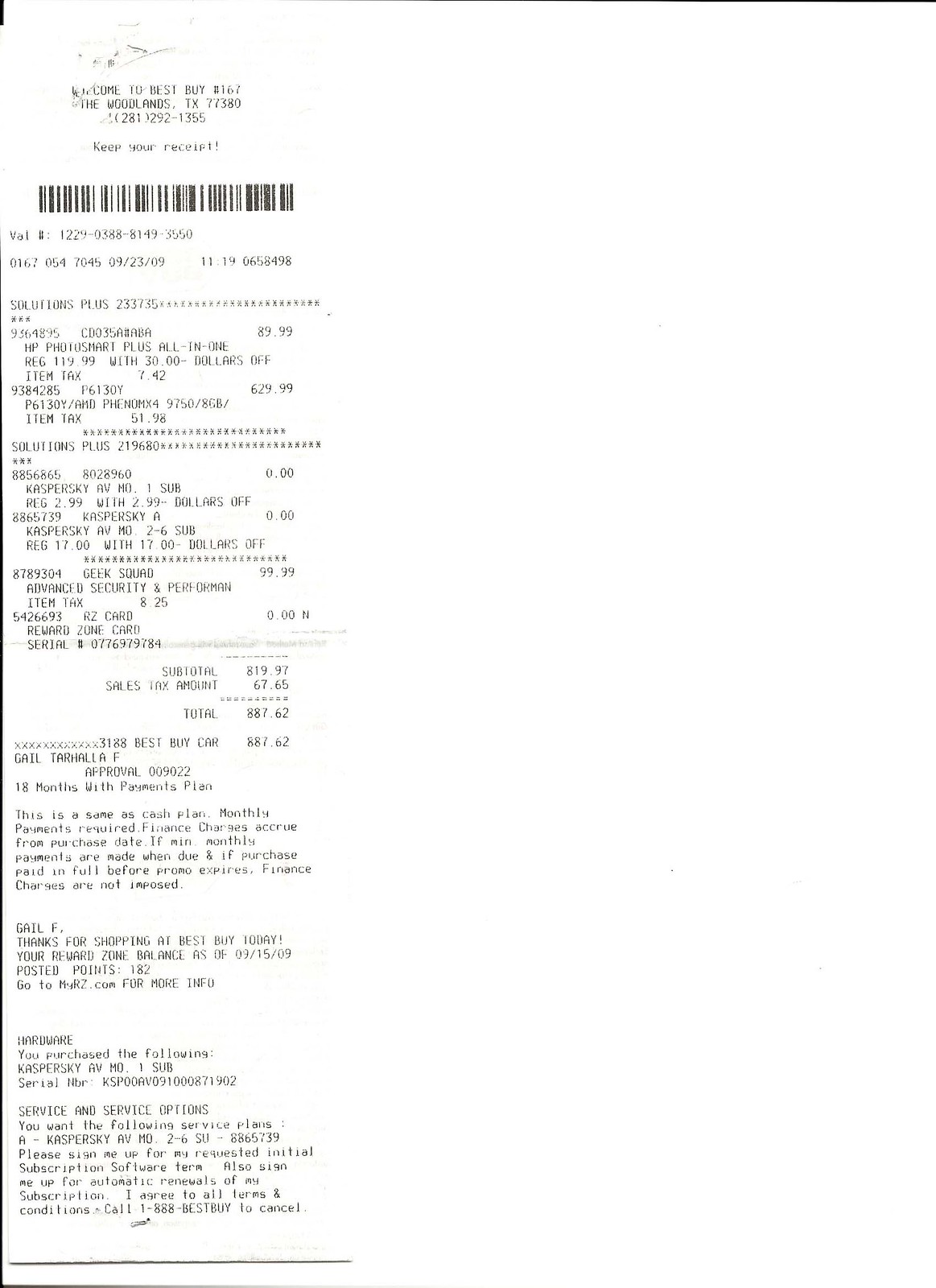This black and white image resembles a low-quality photocopy, possibly of a receipt or a bill. The background is stark white with a thin black line at the top that doesn't span the entire width of the page. On the left side, an elongated object, likely a receipt, is partially visible, with its top edge cut off. About two inches down from the top left corner, the receipt becomes fully visible, stretching all the way down to the bottom and extending slightly into the bottom right corner before fading out.

The receipt is marred by scratches, which have been transferred onto the photocopy. A clearly defined barcode is seen at the top, followed by several lines of black text that are unreadable. A list of items and corresponding charges are evident, suggesting it is a billing statement. In the center of the receipt, a total amount is indicated but is too small to be deciphered. The bottom section contains several paragraphs of text, culminating in another black line below it that touches the bottom edge of the page.